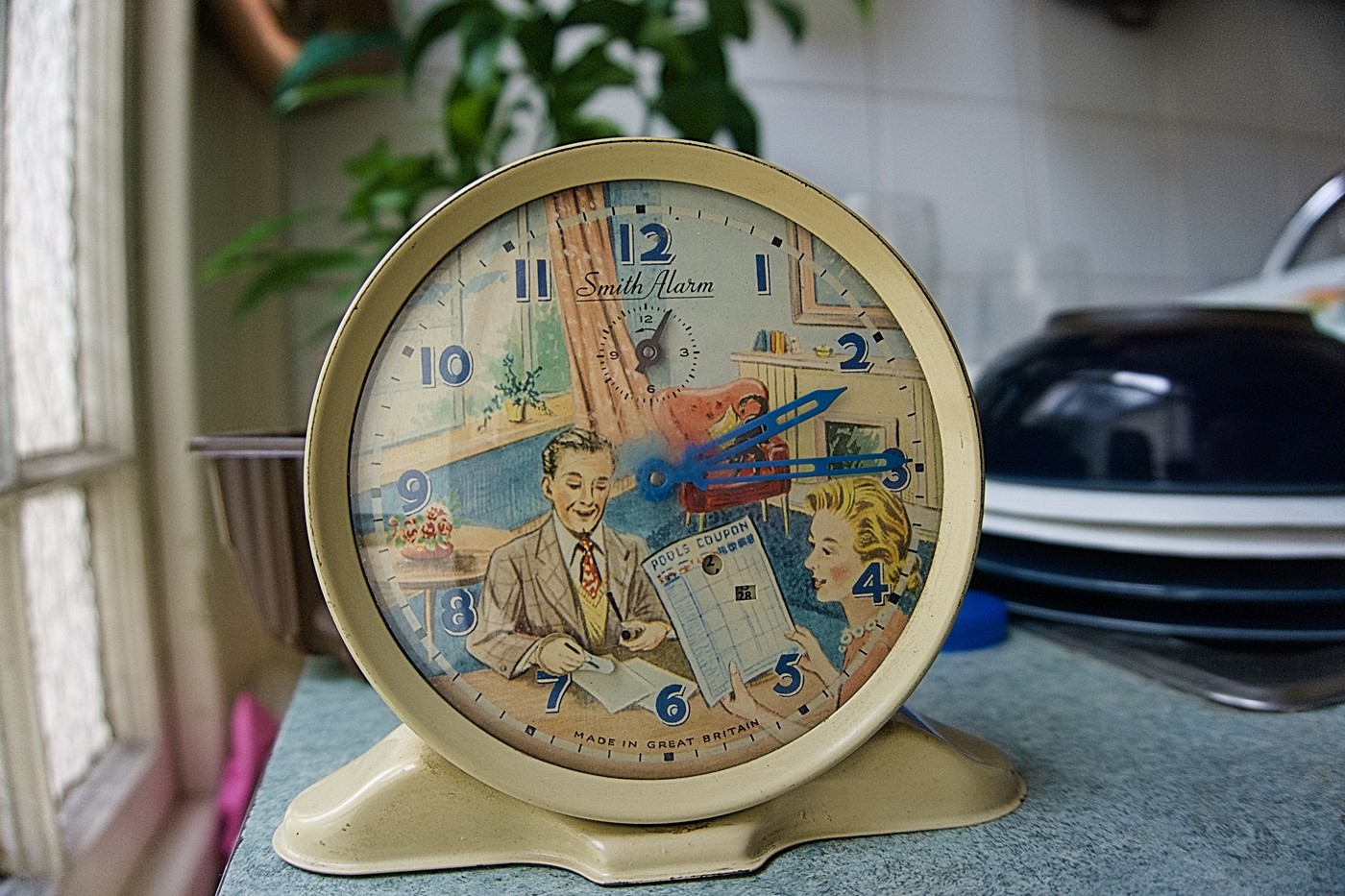This photograph showcases a close-up of a retro-styled clock, prominently placed on what seems to be a kitchen tabletop with a greenish-gray hue. The clock, possibly an advertisement, combines vintage charm with modern design, featuring a light beige, almost metallic finish that gives it a dated yet stylish look. Its face is adorned with a whimsical illustration of a 1950s-era husband and wife, the man dressed in a three-piece suit with a smoking accessory, and the woman involved in a coupon search. The scene encapsulates an Art Deco ambiance with light pastel colors.

Surrounding the clock, the setting includes various kitchen elements: dishes, a sink on the right side, tiles on the wall, and a couple of potted plants behind the clock. The left-hand corner reveals a window with curtains, further enhancing the cozy, domestic scene. Small miscellaneous items scattered in the background add to the lived-in feel, reinforcing the clock's appeal as a charming addition to any household décor.